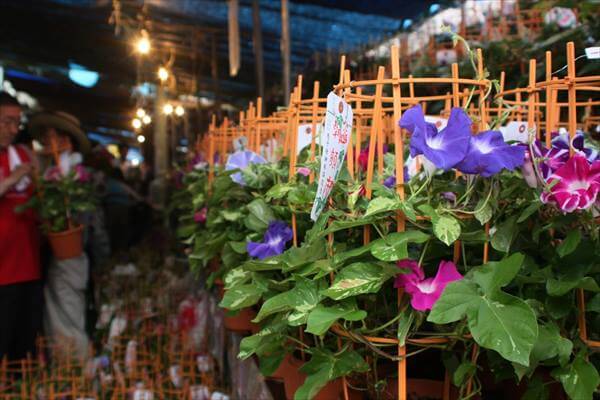This detailed rectangular image, primarily showcasing what appears to be the interior of a greenhouse, presents a vibrant array of petunia plants lined up on a shelf or table in the foreground. These plants boast lush green leaves and radiant blossoms in shades of magenta, pink, and deep purple. Each plant is supported by a cylindrical, wicker-like cage, resembling tomato cages, which are likely made from thin bamboo. Above the plants, there are white tags featuring designs or possibly Chinese lettering. 

In the dimly lit background, the scene shifts to reveal a bustling area where two individuals, one wearing glasses and the other a hat, are engaged with the plants, picking out a pot of flowers from the ground below. Strings of hanging lights, attached to what seems to be a blue tarp ceiling, softly illuminate the space, enhancing the photo's atmosphere. The far left side of the image features more plants in similar cages placed on the ground, while the far right side fades into a darker backdrop, hinting at nighttime, against which a few more red-shirted people can be faintly seen, adding a sense of depth and context to the greenhouse setting.